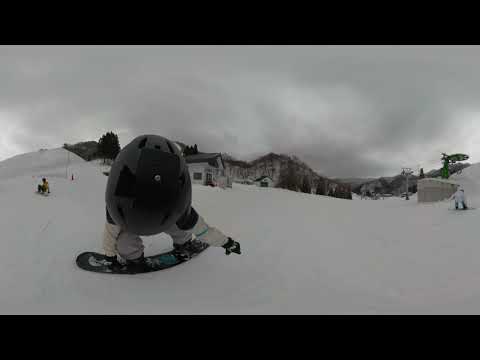In this photograph, a snowboarder dressed in a white suit is captured against a snowy hillside. He is bent over so significantly that his black helmet dominates the frame, making it initially appear as though a black egg or head is riding the snowboard on its own. Upon closer inspection, it's clear he is crouched forward, revealing the perspective. The scene is set on a snow-covered slope with a cloudy gray sky overhead, giving a cold and overcast atmosphere. Behind the main snowboarder, other people can be seen snowboarding as well. In the middle of the image, there is a small white ski building with a black roof, typical of those found on ski slopes. Further in the background, the snowy landscape stretches out, with mountain regions framing the trail and additional snowboarding tracks visible. A ski lift or similar equipment is faintly seen on the right-hand side of the picture, and the photo itself has a dark black border on the top and bottom, adding to its framed appearance.